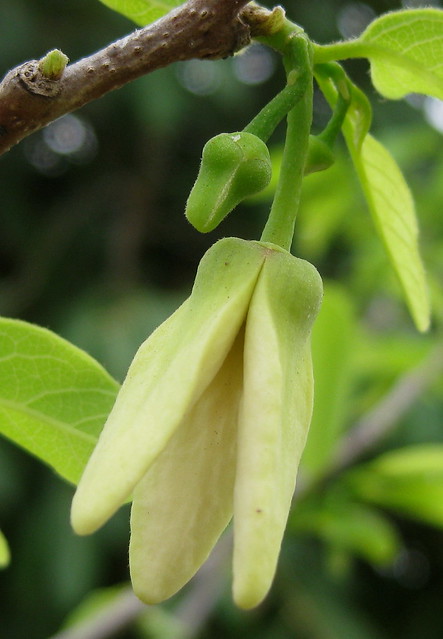A close-up shot of a budding plant captures the intricate details of nature's renewal. The main focus of the image is a branch adorned with vibrant green buds and leaves, highlighting a moment of growth. At the top of the branch, a prominent bud is shown in the process of opening, revealing delicate petals in a lemon meringue hue and three green leaves. The background remains blurred, emphasizing the freshness and vivid coloration of the plant. Although the exact species of the plant is uncertain, the detailed and colorful display suggests it may be located in a natural forest setting or a meticulously cared-for indoor garden.